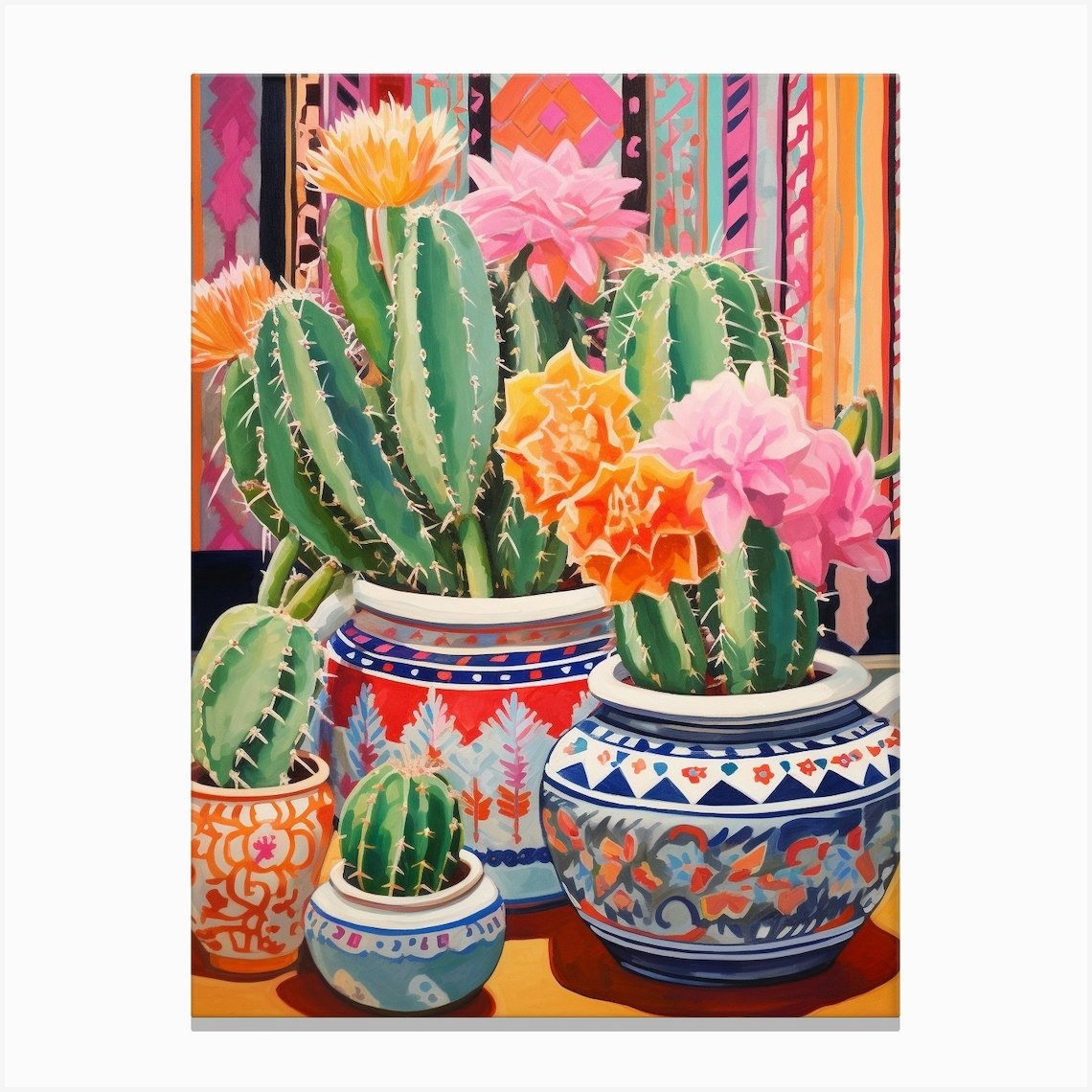This vibrant and detailed painting features a collection of beautifully decorated pottery planters, each housing a unique cactus. In the foreground, a small light teal pot with a blue circle at the top contains a green cactus adorned with yellow spikes. Adjacent to it, a slightly taller pot with an orange-lined white background supports a similarly charming cactus. Moving rightward, a medium-sized pot decorated with blue triangles and pretty floral patterns holds a blooming cactus displaying yellow and pink flowers. Dominating the scene is the largest pot at the back, adorned with images of trees shaded in orange, pink, and white, set against a striped background. This planter contains the most flourishing cactus, with multiple orange and pink blossoms. The background of the painting adds to the lively atmosphere with its colorful, abstract vertical lines in shades of orange and pink, enhancing the overall cheerful and dynamic feeling of the artwork.